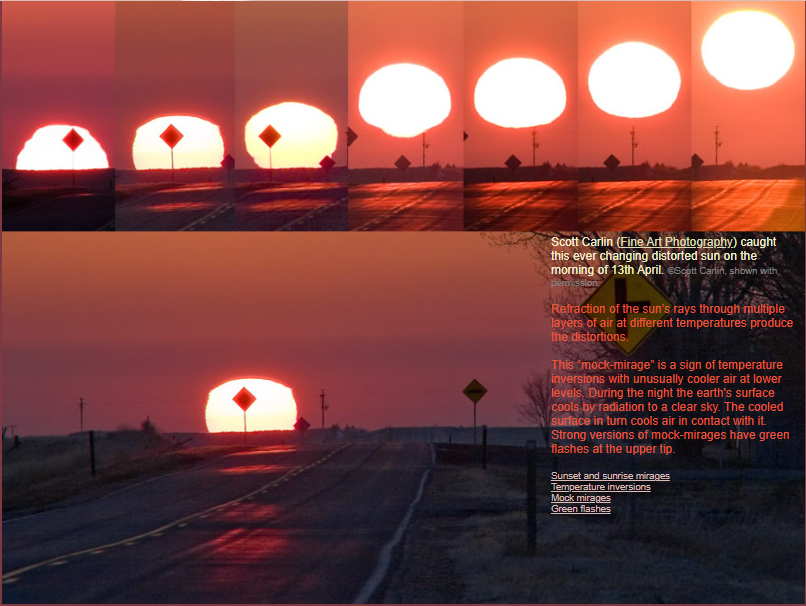This almost square-shaped image features a horizontally aligned rectangular composition at the top, consisting of seven vertical rectangles illustrating the progressive rise of the sun. Each rectangle showcases a road and a diamond-shaped road sign while the sun ascends from just above the horizon on the far left to the top of the frame on the far right. All of these segments share a pink sky backdrop. Below these smaller panels is a larger horizontal rectangular picture, appearing to be a close-up of the second panel from the top row. On the right side of the image, text reads: "Scott Carlin Fine Art Photography caught this ever-changing distorted sun on the morning of 13th April. Refraction of the sun's rays through multiple layers of air at different temperatures produced the distortions. This mock mirage is a sign of temperature inversions with unusually cooler air at lower levels. During the night, the Earth's surface cools by radiation to a clear sky. The cooled surface, in turn, cools air in contact with it. Strong versions of mock mirages have green flashes at the upper tip."